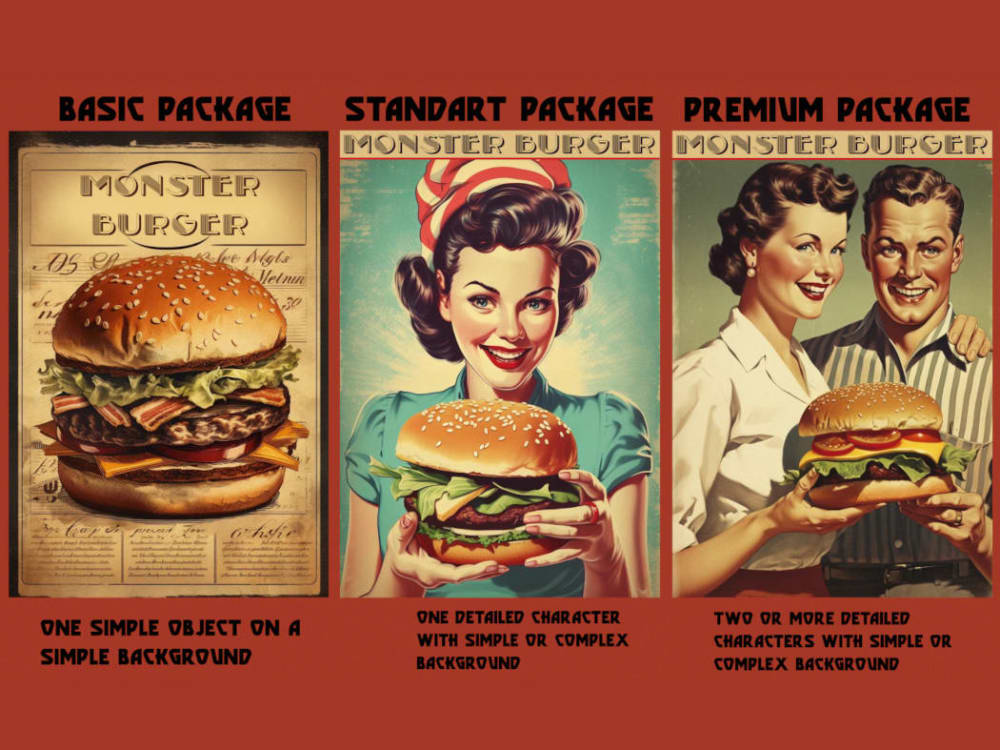The image is a vintage-style, full-color digital pricing graphic for a graphic artist’s service packages, set against a red background. There is no border. The display consists of three horizontally arranged images, each representing a different service package. 

On the left, labeled "Basic Package," there is an image of a cheeseburger named "Monster Burger." The accompanying text reads "One Simple Object on a Simple Background." The middle image, labeled the "Standard Package," features a woman dressed in a blue top and a red-and-white striped hat, holding a cheeseburger. The text below this image states "One Detailed Character with Simple or Complex Background." The rightmost image, the "Premium Package," shows a man and a woman together holding up a large cheeseburger, with text below that reads "Two or More Detailed Characters with Simple or Complex Background." The overall aesthetic suggests a 1940s or 1950s era theme.